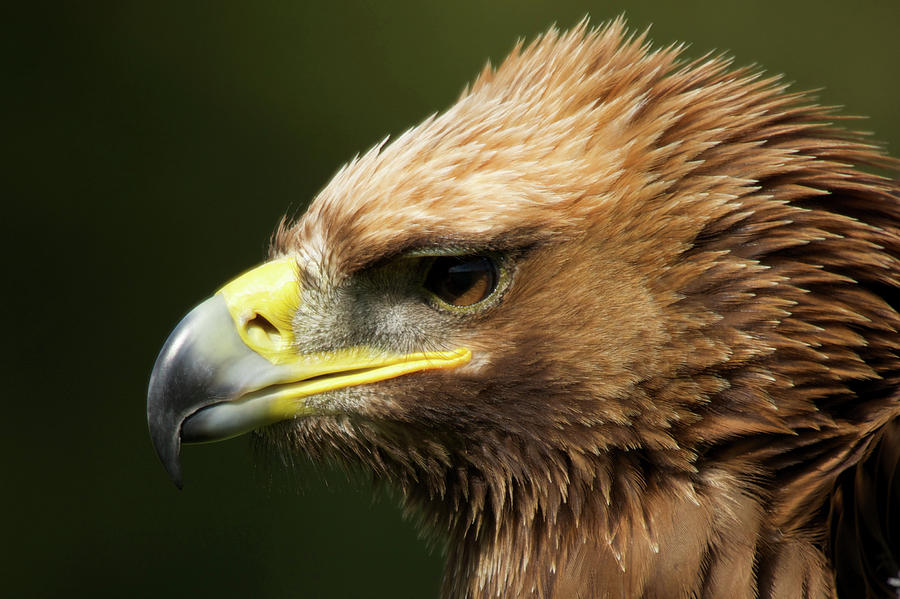This close-up photograph captures the intense profile of a young eagle, focussing on its face and upper neck. The bird's predominantly brown feathers flow backwards, tipped with white for additional texture, becoming creamier at the top of its head. Sparse feathers around the beak reveal grayish skin, while the area above the head has more white spotting. The eagle's sharp, hooked beak transitions from a bright yellow at the nostrils to a gradient of gray, ending in a nearly black tip. Its large nostrils are prominently visible. The eagle's eye, with a brown iris and heavy eyelid, adds to the bird's fierce expression. The blurred background in shades of gray and black ensures that the majestic details of the eagle remain the main focus of the image.